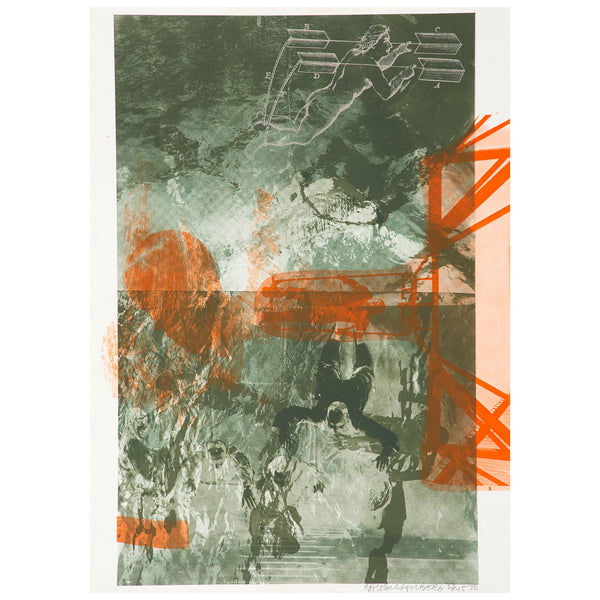The image is a detailed painting or drawing on canvassed paper, primarily designed in shades of green with distinct orange and white accents. This vertical rectangular artwork features an intricate depiction of an angel at the top, outlined in white, appearing to fly with arrows emerging from its arms and back. The background is a mix of dark green smudges, lending an overall abstract feel to the piece. Around the center, bright orange splatters are interspersed with vertical and horizontal lines, adding a sense of chaotic motion. Below, the scene includes a man seemingly jumping face-first towards the ground, surrounded by other vaguely defined figures in green and orange hues, creating an impression of movement and urgency as they scatter or run away. The abstract nature of the painting makes some elements hard to discern, contributing to its mysterious allure.